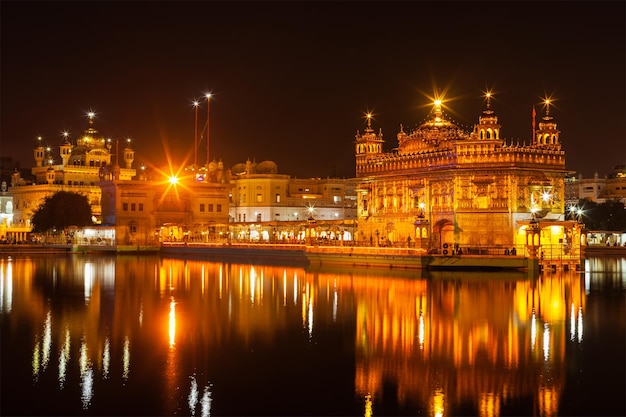This image is a vibrant and mesmerizing night scene featuring a still waterfront that occupies the bottom third of the frame. The glassy, dark water serves as a perfect mirror, reflecting the illuminated skyline above. The skyline consists of intricately decorated, ornate buildings that evoke European or possibly South Asian architecture. These structures are likely made of stone or concrete blocks and are bathed in warm yellow-golden lights, creating an almost magical, glowing effect. The buildings give the impression of being placed on a small dock or pier that juts into the water. 

Above this illuminated block, the sky is a deep black, subtly tinged with a small aura of light pollution, fading into a lighter purple hue. One bright light crowns a particularly tall, intricately ornamented building, while another bright light is situated to the left side of the image. The detailed terraces and possible relief work on the buildings enhance their opulent appearance, making the scene feel almost royal. The stillness of the water and the absence of boats or visible people add a serene and almost surreal quality to the scene. A well-manicured tree can be seen next to one of the buildings, contributing to the overall charm of this beautifully lit nighttime waterfront.